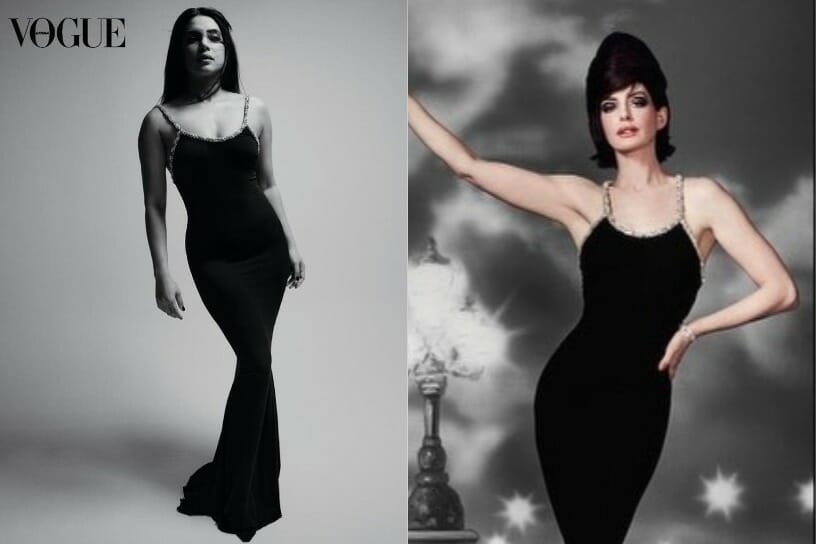The image displays two Vogue magazine covers side-by-side, both featuring prominent actresses in striking, black, form-fitting evening dresses with spaghetti straps. The photo on the left is in black and white, presenting Indian actress Priyanka Chopra elegantly posing with her legs crossed and slightly bent, accentuating the dress's body-hugging design. Her long, dark hair cascades down her back, and the iconic black Vogue logo is positioned in the top left corner.

On the right, the image appears to blend black and white with subtle colorization, particularly highlighting the Caucasian skin tone of the actress, who is identified as Anne Hathaway. She wears an identical dress and sports a glamorous, vintage 50s or 60s bouffant hairstyle. Anne poses with her right hand raised and her left hand resting on her hip, alongside a retro-style street lamp in the background. Both photographs evoke a classic, timeless elegance, characteristic of Vogue magazine's sophisticated fashion presentations.